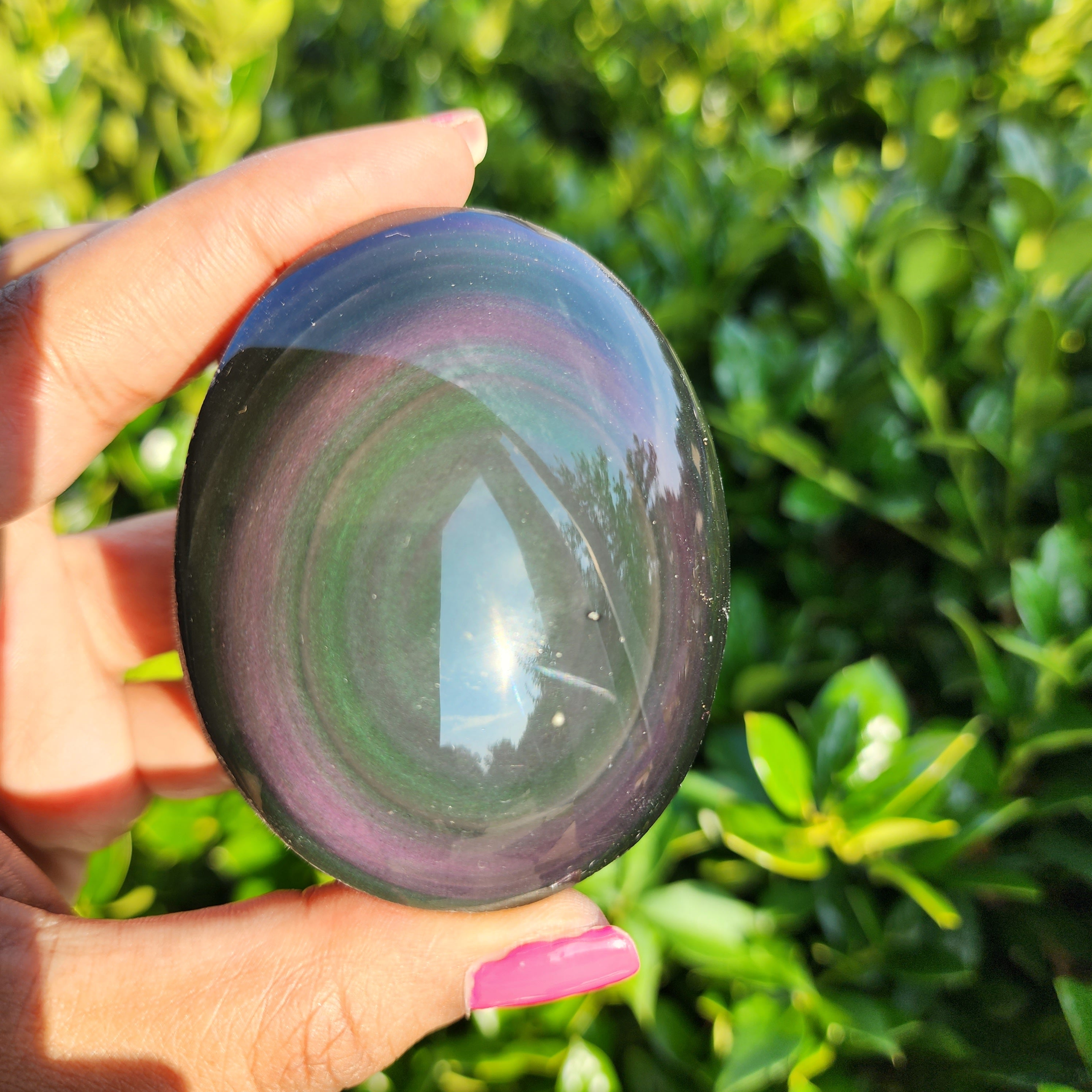In the image, a woman's hand, with long nails painted a bright pink, delicately holds a large, oval gemstone between her thumb and index finger. The gemstone is highly polished and glossy, catching the sunlight and reflecting blue skies. The stone is predominantly gray in the center, featuring a faint green swirl and a purplish bar that resembles a brushstroke. The edges of the gemstone darken to deep green and blue hues. Surrounding the hand, the blurred background reveals green and yellow waxy bushes, adding to the serene, natural setting.